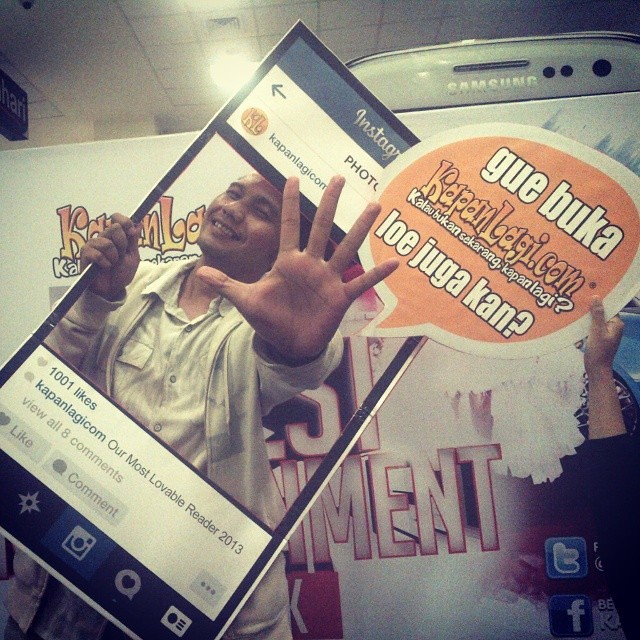In this vibrant event photo, an Indonesian man joyfully poses with a life-sized Instagram frame cutout, mimicking a social media post. He holds the frame in his left hand, while his right hand playfully emerges through the cutout, positioned as if signaling "stop." He is smiling and winking at the camera, creating an inviting and engaging expression. The Instagram frame showcases the user "Kapanlagicom" and highlights "1001 likes" along with the caption "Our most lovable reader 2013." Notably, there are small Twitter and Facebook logos located at the bottom right of the frame. Behind him looms a giant Samsung phone as part of a promotional backdrop with a large board containing some text. Additionally, an orange speech bubble with a white outline, bearing text in a foreign language, adds an extra layer of visual interest.